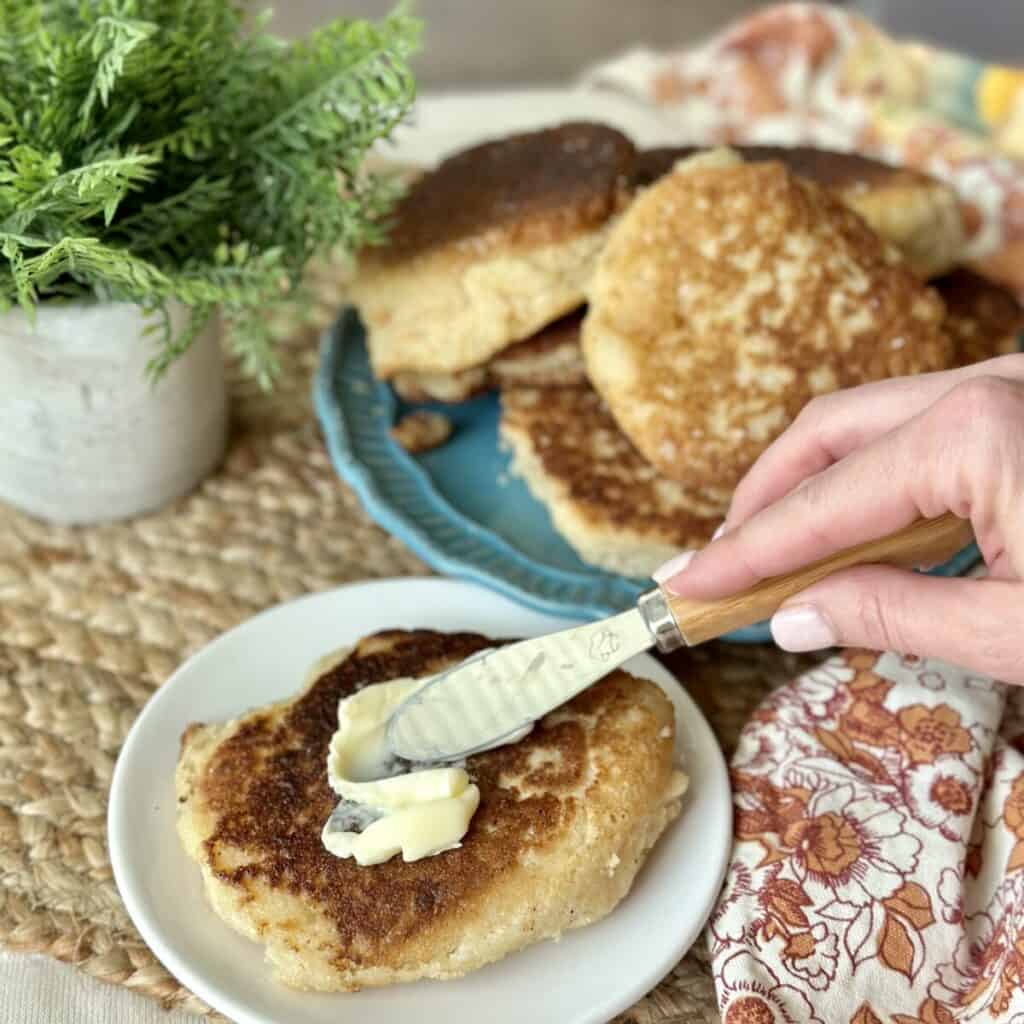In this photo, we see a left hand with white nail polish, holding a butter knife with a wooden handle, spreading butter onto a slightly burnt pancake on a white plate. The scene is set on a brown woven table runner. In the foreground, the white plate rests above a white napkin adorned with orange and maroon floral designs. To the right of this plate, partially visible, is a blue plate stacked with more pancakes. In the background to the left, there is a ceramic pot containing an artificial fern. The focus is primarily on the hand buttering the pancake, with the background elements somewhat blurred, emphasizing the detailed action in the foreground.